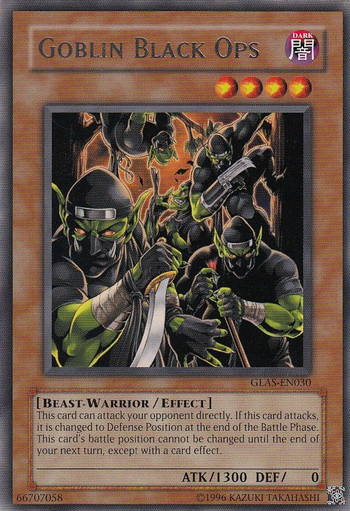The image depicts a detailed portrait-oriented Yu-Gi-Oh! trading card, prominently featuring six or more muscular green goblins adorned in gray armor helmets and wielding various weapons such as swords, knives, claws, and staffs. These goblins are aggressively charging towards the viewer. The background of the card is black, and the illustration is encased within a gray border. At the very top of the card, it reads "Goblin Black Ops" in black text, accompanied by a circular logo with Japanese characters. Directly underneath are four red circles, each containing a yellow star. The bottom section features a light brown background with black text stating "Beast-Warrior-Effect." The card's effect is described as follows: "This card can attack your opponent directly. If this card attacks, it is changed to defense position at the end of the battle phase. This card's battle position cannot be changed until the end of your next turn except with a card effect." The card's stats are marked with "ATK/1300, DEF/0." There are also small, nearly illegible numbers and letters, including a copyright marking from 1996 attributed to Kazuki. This card is a single object that dominates the entirety of the photograph, displaying a mixture of colors like red, purple, white, tan, silver, orange, black, green, gold, and yellow, which suggests its use in a strategic trading card game like Yu-Gi-Oh!